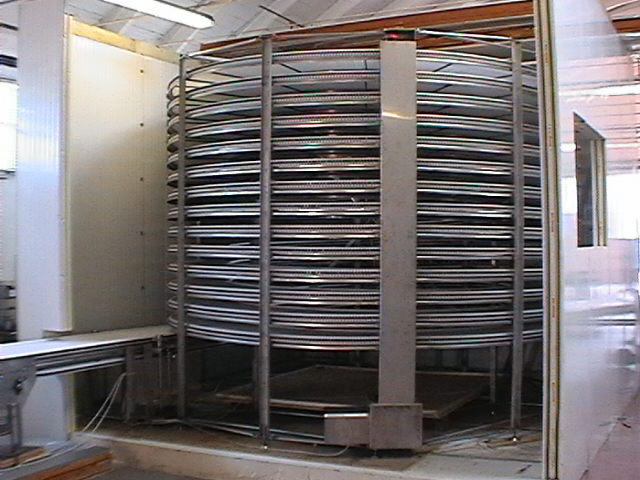This photograph captures a complex industrial machine inside a factory. The machine is circular with multiple layers of steel discs, resembling large Frisbees or trays, with an overall height of approximately 15 feet. It features a prominent metal pole running through the center, anchored by an electric motor and adorned with a red light at its apex. The structure is supported by steel beams and is housed within a room flanked by light brown or off-white walls. There is also wood reinforcement visible at the top left, a makeshift square window on the right, and a reflective surface catching light from the factory’s ambient lighting. To the bottom left, a conveyor belt feeds materials into the machine, suggesting that it processes these inputs. The room’s roof appears to be adjustable, indicating potential flexibility in operations. Overhead, vertical fluorescent lighting illuminates the intricate setup.